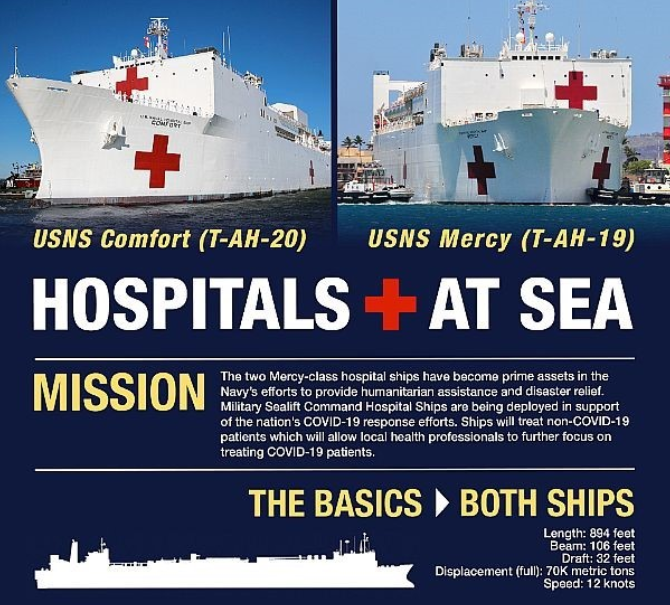This poster serves as an informative advertisement about the US Navy's hospital ships, USNS Comfort (T-AH-20) and USNS Mercy (T-AH-19). Predominantly white with large red crosses adorning their sides and superstructures, these Mercy-class hospital ships are described as crucial assets in delivering humanitarian assistance and disaster relief globally. 

At the top of the poster, there are two side-by-side images of these colossal medical vessels: USNS Comfort on the left and USNS Mercy on the right. The poster's centerpiece is the title "Hospitals at Sea," prominently displayed in white letters against a dark blue background, with a red medical symbol nestled between the words. Below, there is detailed text that highlights the ships' missions, emphasizing their role in treating non-COVID patients during the COVID-19 pandemic to free up onshore facilities for critical cases and prevent the spread of the virus.

Additionally, the poster includes specific technical data about the ships, such as their diameter, length, displacement, and speed, along with a simplistic, cartoonish silhouette of the vessels in the bottom left corner. Through well-coordinated text and visuals, the poster underscores the significant contribution of these floating hospitals in international medical relief efforts, demonstrating their capability to travel anywhere needed to provide a comforting, hospital-like environment at sea.